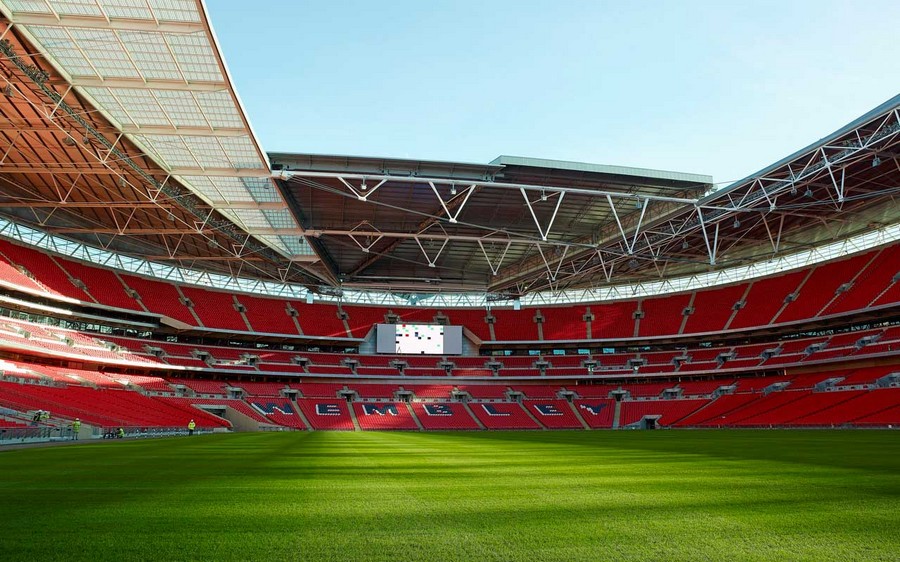This photograph captures the iconic Wembley Stadium in the UK from one end of the pitch, providing a sweeping view of the venue. The focal point is the opposite end, where the word "WEMBLEY" is clearly spelled out in black and white seats amidst a sea of predominantly red seating. The vibrant green soccer pitch glistens under the natural light, with subtle shadows cast by the partially open roof, hinting at the clear blue sky above. To the left, a group of four or five individuals in bright yellow-green reflective jackets can be seen in the distance, likely groundskeepers or staff preparing for an upcoming game. The scoreboard, situated in the background, displays a blank white screen with scattered red, black, and green squares, adding a touch of modernity to the historic site. The overall ambiance is serene and orderly, embodying the calm before the electrifying energy that a game day brings.